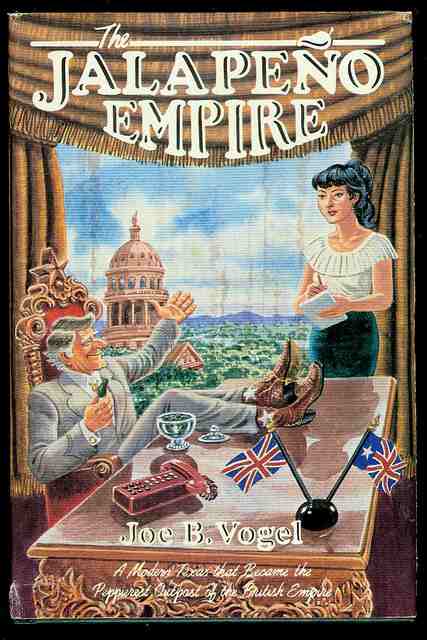The image depicts the cover of a book titled "The Jalapeno Empire" by Joe B. Vogel. At the top of the cover, the title is prominently displayed in white, with a small white jalapeno icon and a line cutting through the word "The." The scene features an authoritative man seated comfortably at a desk, which has a smooth, shiny, brown surface. This man, clad in a gray suit and sporting gray hair, has his feet propped up on the desk, revealing cowboy boots adorned with white stars. He appears to be enjoying a drink, possibly champagne. The man sits in an ornate, red throne-like chair with a golden star at the top. Standing beside him is a woman, likely his secretary, with brown or black hair and dressed in a white shirt. She is writing on a notepad, presumably taking dictation from the man. The desk is decorated with two British flags and an old-fashioned red telephone. In the background, there are blue and white curtains framing a window, through which a Capitol building, likely in Texas, is visible. The bottom of the cover contains additional text in cursive, describing "a modern Texas that became the outpost of the British Empire," although the exact wording is hard to read. Overall, the cover conveys a theme of power and imperial reach, blending elements of Texas and British iconography.